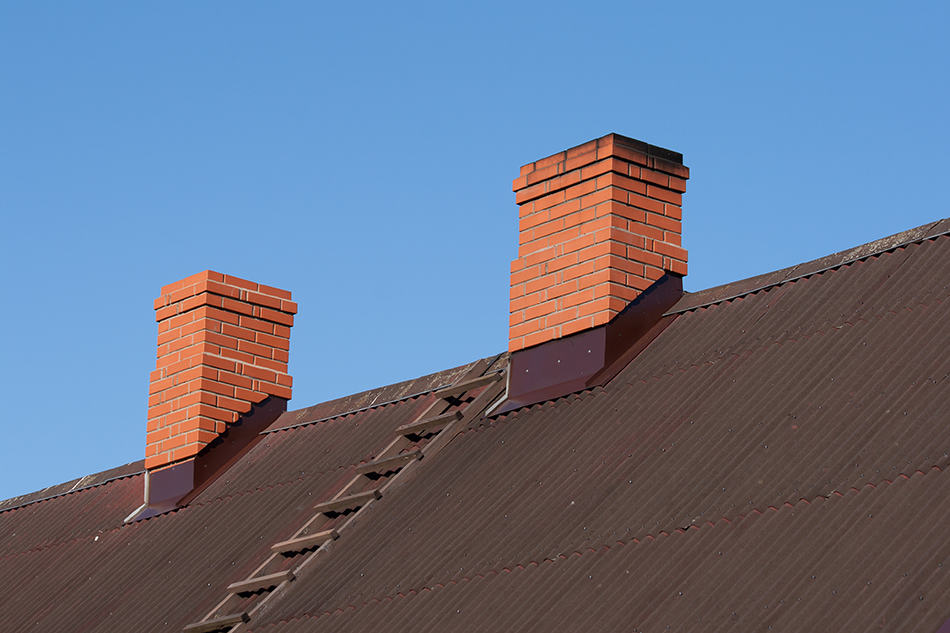The image showcases the sharply slanted roof of a building under a brilliantly clear, blue sky that occupies the top half of the picture. At the highest point, the roof slopes down from right to left and is covered in dark brown corrugated metal sheets, suggesting rust with age. Prominently, two brick chimneys are positioned along the roof, with the first chimney starting around 15% from the left edge and the second one around 55%. The chimneys, a few feet apart, each have a metal base extending about six inches up. The right-hand chimney shows signs of use, marked by blackened bricks near the top. Between the chimneys, closer to the one on the right, a wooden ladder with rails is built into the roof, leading up toward the peak.